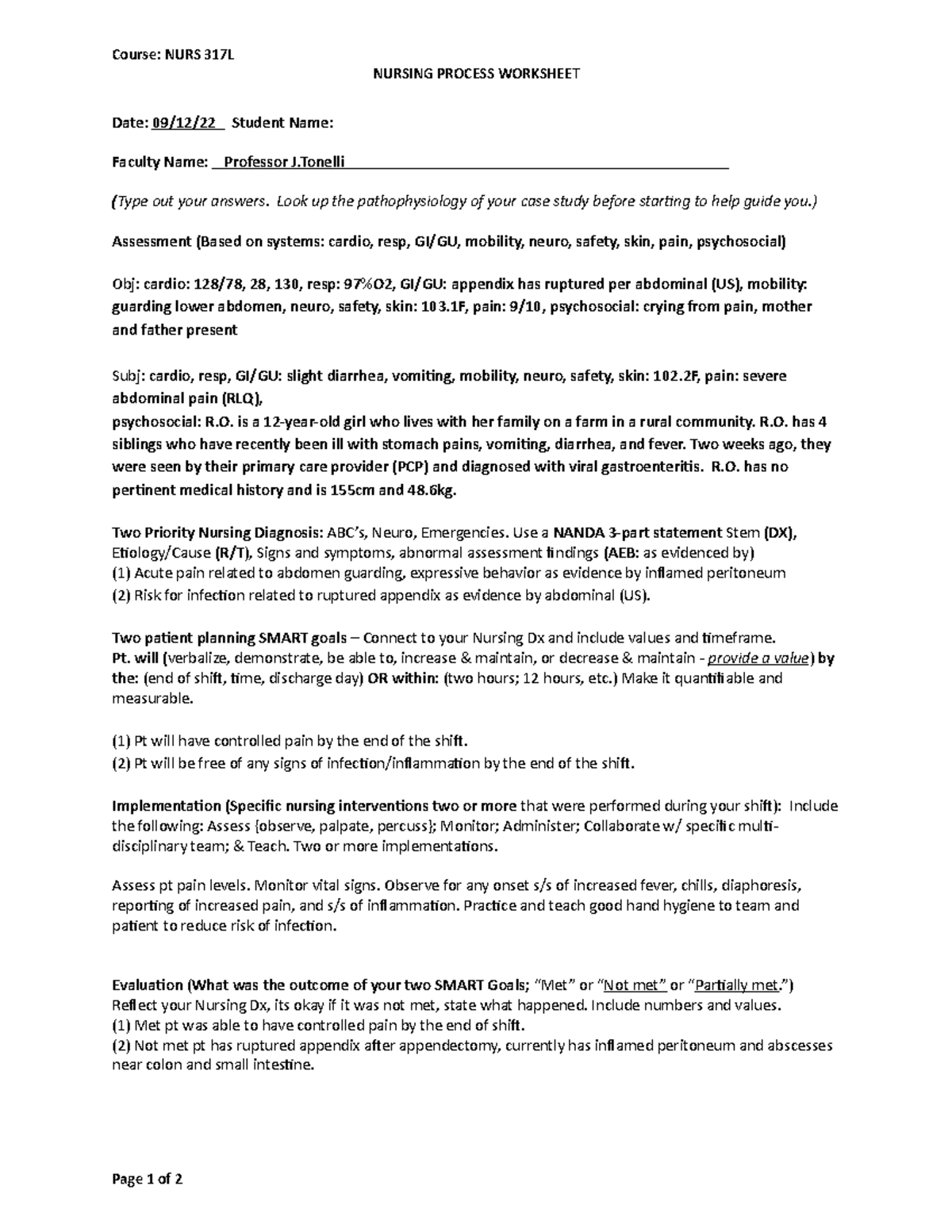**Detailed Caption:**

The image displays a "Nursing Process Worksheet" against a black and white background with black text. At the top, it reads "Course: NURS317L" and is titled "Nursing Process Worksheet" dated "09-12-22." The student is required to fill in their name along with the faculty name, specified as "Professor J. Tonelli."

Below the header, instructions prompt students to research the pathophysiology of their case study before beginning the worksheet for guidance. Key sections are highlighted in bold for clarity and include:

- **Assessment Based on Symptoms**:
  - **Cardio**: Blood pressure 128/78 mmHg, heart rate 130 bpm.
  - **Resp**: Respiration rate 28 breaths/min, oxygen saturation 97%.
  - **GI/GU**: Appendix rupture confirmed via abdominal ultrasound.
  - **Mobility**: Guarding of lower abdomen observed.
  - **Neurosafety**: Not specified in detail.
  - **Skin**: Temperature recorded at 103.1°F.
  - **Pain**: Rated as 9 out of 10.
  - **Psychosocial**: Patient is crying from pain, with both mother and father present.

Further details include additional symptom assessment:
  - **Cardio**: No new data.
  - **Resp**: No new data.
  - **GI/GU**: Reports slight diarrhea and vomiting.
  - **Mobility**: No new data.
  - **Neurosafety**: No new data.
  - **Skin**: Temperature recorded at 102.2°F.
  - **Pain**: Severe abdominal pain located in the right lower quadrant (RLQ).
  - **Psychosocial**: RO is a 12-year-old girl living with her family on a farm in a rural area. She has four siblings who recently experienced stomach pains, vomiting, diarrhea, and fever, all diagnosed with viral gastroenteritis by their primary care physician (PCP). RO herself has no pertinent medical history and measures 155 cm in height and weighs 48.6 kg.

At the bottom, sections for "Diagnosis," "SMART Goals," "Implementation," and "Evaluation" are outlined but not filled in.